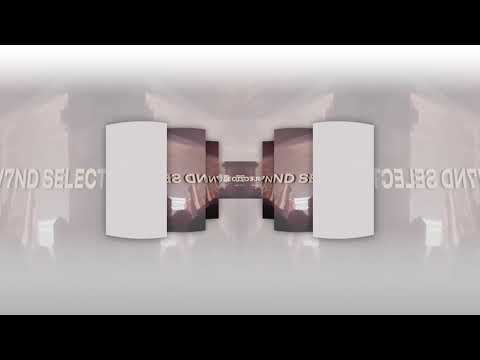The image is a slightly bewildering visual, featuring random and indistinct elements. Central to the image is a set of repeated white words reading "7ND Select," which appear mirrored on each side of the picture. The overall composition suggests a vertical rectangular picture framed by horizontal black stripes on the top and bottom. At the center lies a shiny, reflective white surface dotted with several rectangular shapes. These rectangles are situated symmetrically, with three on each side, gradually aligning towards the center in a mirrored arrangement. The closest rectangles are solid white, while the further ones exhibit an indiscernible, pinkish-hued image that remains unclear even when scrutinized. The entire image is enveloped in a blurry, foggy effect, further obscuring any discernible details and creating a challenging experience in identifying specific objects or figures within the photographs embedded in the composition.